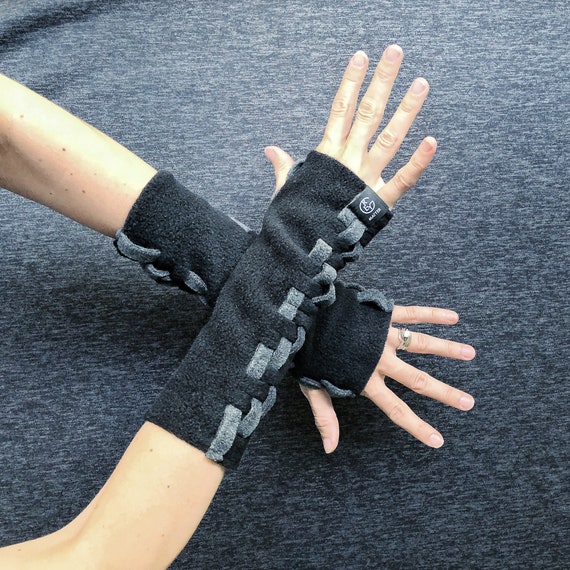This photograph captures the forearms of a light-skinned woman, identifiable by an engagement ring and manicured fingernails on her left hand. Her forearms stretch from the left side of the frame and cross at the wrists, forming an X-shape with her fingers extended. The forearms are adorned with dark gray woolen or felt fabric arm warmers, extending from mid-forearm to the base of the fingers, with thumb holes for a secure fit. The arm warmers feature a pattern of interwoven lighter gray stitching and possibly a lighter strip of felt. Although there is a logo tag on the right arm warmer, it remains unreadable. The backdrop of the image is a lighter gray, possibly speckled or fabric material, adding to the overall composition.